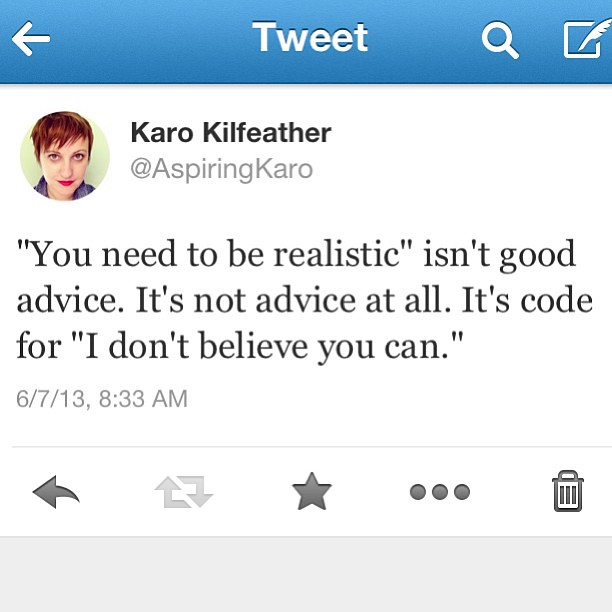The image is a screen grab from a phone featuring a social media post on Twitter. At the top of the screen, there's a blue banner that spans the width of the image. On the left side of this banner, there's a white arrow pointing left. In the center of the banner, the word "Tweet" is displayed in white text. Adjacent to it is a stylized white cartoon magnifying glass, followed by a square icon with a feather quill on the right side.

Beneath this banner is the profile information and tweet content. The profile picture shows a woman with short, reddish-brown hair and red lipstick, gazing slightly upwards. To the right of this image, the display name reads "Kara Killfeather," followed by the handle "@AspiringKaro." The tweet text says, "You need to be realistic isn't good advice. It's not advice at all. It's code for I don't believe you can." Below the tweet, the timestamp reads "8/7/13, 8:33 AM."

At the bottom of the image, there are various icons: a go back arrow to the left, a star next to it, three dots further to the right, the retweet symbol depicted as up and down arrows in a loop, and finally, an image of a trash can on the far right.